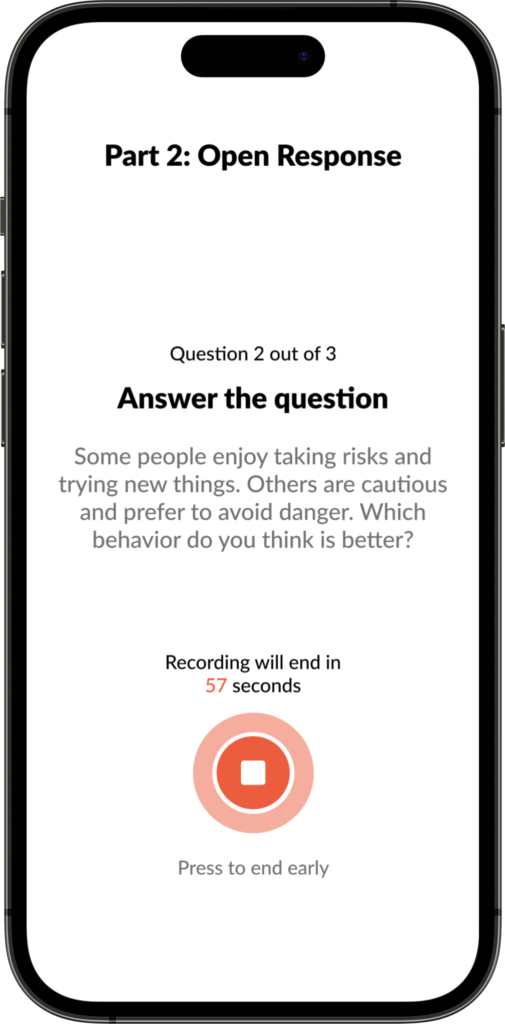The image displays a sleek, modern UI UX design of a newer model iPhone, characterized by its elegant black outline and distinctive features. At the top of the phone is a small black bar housing the front camera. The right side of the phone features a prominent lock screen button, while the left side hosts two volume buttons and a smaller button for toggling sound on and off.

The entire screen of the phone is rendered in white, providing a clean and minimalist backdrop. Prominently displayed at the top is the title "Part Two: Open Response" in large, bold letters. In the center of the screen, there's a prompt stating "Question 2 of 3: Answer the question," followed by the query, "Some people enjoy taking risks and trying new things, while others are cautious and prefer to avoid danger. Which behavior do you think is better?"

Below this question, a countdown timer indicates that "Recording will end in 57 seconds," alongside a red circular record button with a square in its center, symbolizing the recording function. At the very bottom of the screen, there's an option labeled "Press to end early," enabling users to conclude their response before the timer runs out.